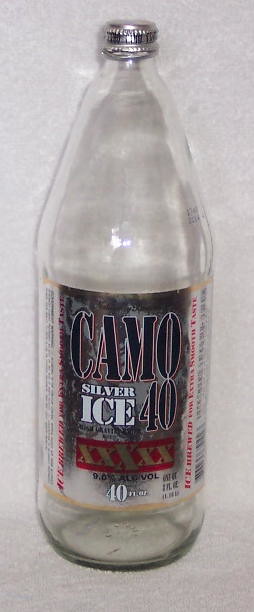The photograph showcases a glass bottle standing upright against a background consisting of a white ground and a white wall. The bottle is clear and topped with a silver metal cap. It is empty and adorned with a partially translucent label that features a mix of black, red, and white colors. The label prominently displays the text "Camo Silver Ice 40," accompanied by five X's. Additional details at the bottom of the label indicate the bottle's capacity as 40 fluid ounces and its alcohol by volume percentage of 9.6. There is also some vertical text on the label, though it is illegible due to the low resolution of the image. A serial number is visible on the side of the bottle, suggesting that it might be a type of beer or malt liquor.